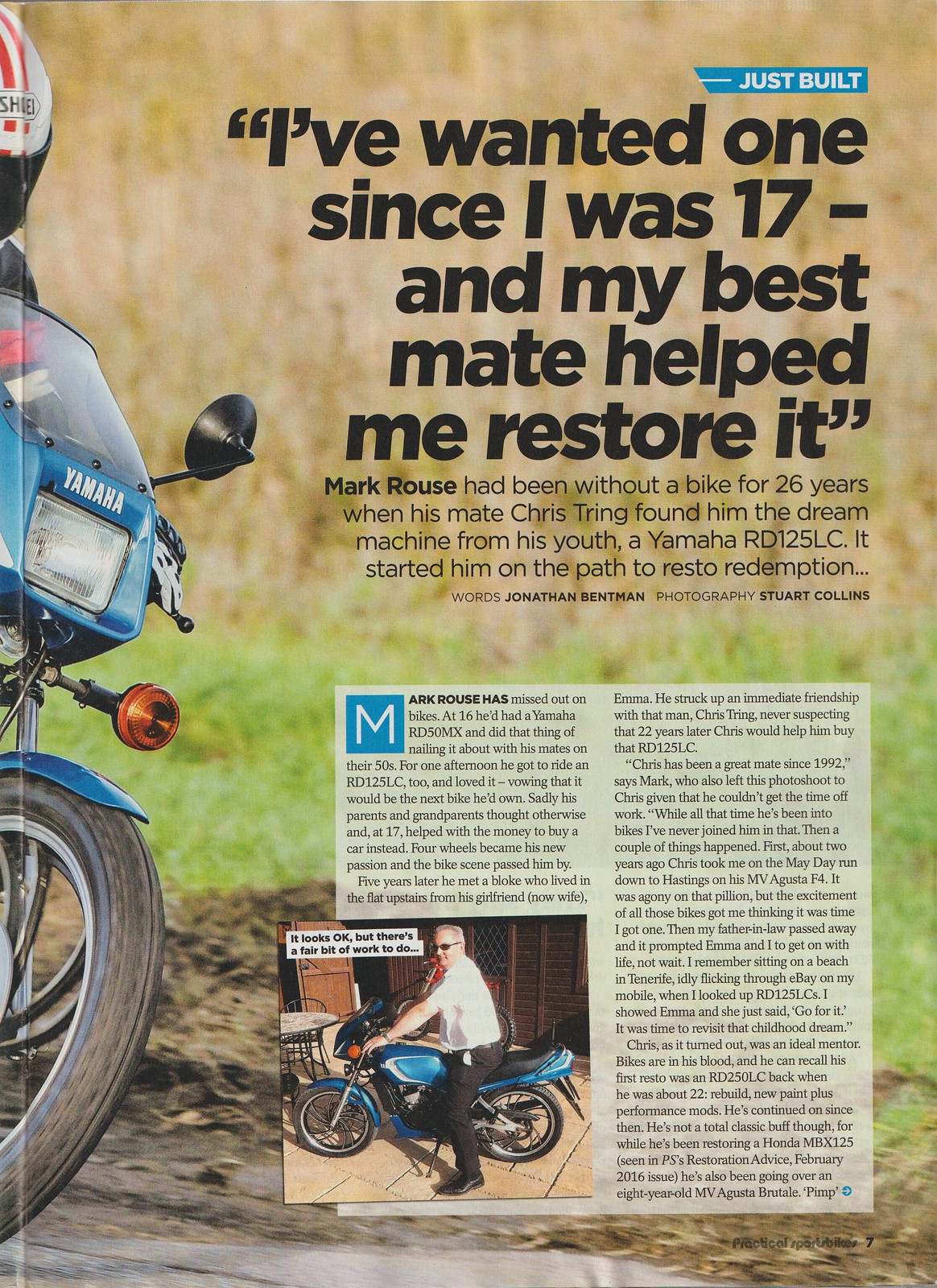The magazine spread from Practical Sports Bikes, page 7, features the journey of Mark Rouse, who had been without a motorcycle for 26 years until his friend Chris Tring helped him restore his dream machine from youth, a Yamaha RD125LC. The title "Just Built" is prominently positioned, with Mark's words, "I've wanted one since I was 17, and my best mate helped me restore it," capturing the sentiment of a long-held desire fulfilled. The image depicts the front part of a bicycle, including the tire, front fender, and windshield, accompanied by a mask or helmet. Beside it, the smaller print details, "Mark Rouse had been without a bike for 26 years when his mate Chris Tring found him the dream machine from his youth, a Yamaha RD125LC. It started him on the path to resto redemption." The article, with words by Jonathan Bentman and photography by Stuart Collins, narrates this story of restoration and the rekindling of a passion for motorbikes. An inset of an article, though small and unreadable, adds depth to the narrative. Below the text, there is a photograph of Mark Rouse himself, a middle-aged Caucasian man dressed in dress pants and a short-sleeved shirt, wearing sunglasses, standing next to his restored, striped blue Yamaha RD125LC.